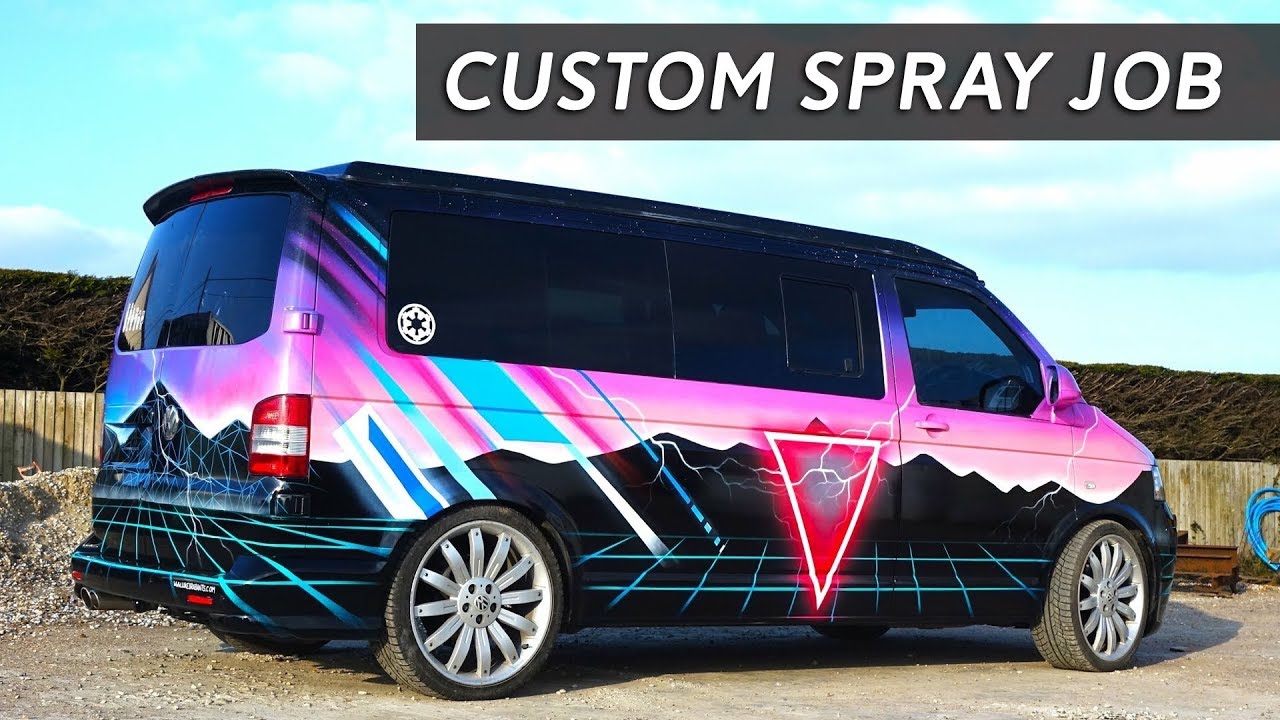This high-quality photograph showcases a van with an intricate custom paint job, prominently featuring in an outdoor setting. The van is parked in a gravel parking lot bordered by a wooden fence, with a clear blue sky dotted with fluffy clouds in the background. A dark gray rectangle overlay in the top right-hand corner of the image displays the words "CUSTOM SPRAY JOB" in bold white letters.

The van's custom artwork is striking: the bottom half is adorned with black-painted mountains overlaid with a blue grid, transitioning to a flat black area featuring a neon greenish-blue grid or reticle. The vibrant upper portion of the van showcases a gradient from pink at the bottom to purple at the top, interspersed with diagonal blue, purple, and white lines toward the rear.

A standout feature on the rear door is an inverted white triangle with red outlines, from which lightning bolts streak from the top right to the bottom left. Adding a touch of fandom, a Star Wars Rebel Alliance sticker is positioned in the right-hand rear window. The van is oriented sideways to the camera, displaying the rear and part of the side, and is equipped with white rims.